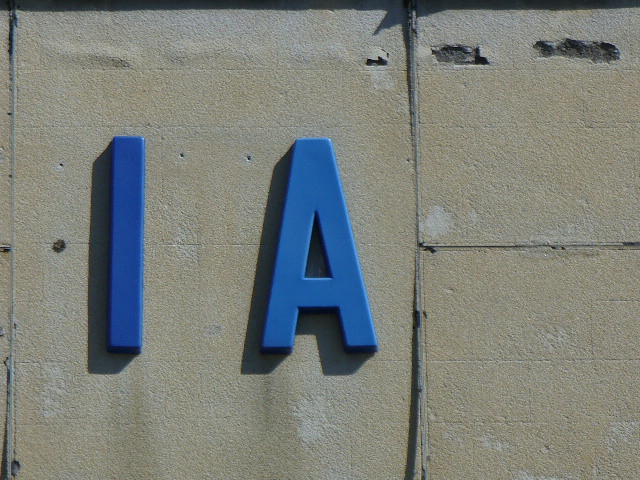The image depicts large, blue letters "I" and "A" prominently positioned against a wall that has the appearance of white bricks that have aged and yellowed over time, resembling the effects of long-term cigarette smoke exposure. The bricks, however, are likely a textured drywall designed to mimic the look of real bricks. This is suggested by the presence of bubbles and swelling near the top of the wall, indicative of water damage typically seen in drywall. A pipe runs vertically down the center of the wall, splitting off to the right halfway down, and there are a few holes in the upper right section of the wall, adding to the impression that the material might be thin brick veneer or drywall.